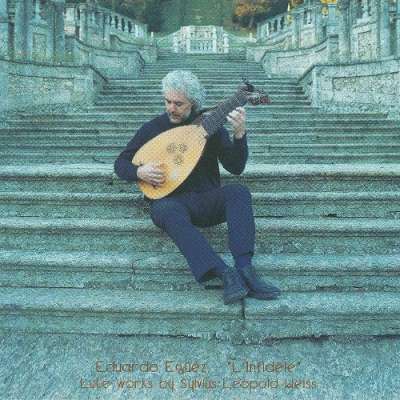In the photograph, an elderly man with curly, silvery-gray hair is seated on a broad stone staircase reminiscent of the Spanish Steps in Rome. He is intently looking at his hands as they dexterously play a light-brown lute. The man, dressed in a black long-sleeved shirt and dark navy slacks paired with black shoes, is centered in the image, drawing the viewer's focus. The background features a historical, weathered stone architecture that adds an artistic, almost melancholic atmosphere to the scene. The colors in the image are dominated by shades of blue, green, white, brown, and tan, giving the photograph a soft, muted tone. At the bottom of the image, barely legible text reads "Eduardo Egüez," followed by "La Infidel" and "Lute Works by Silvius Leopold Weiss," indicating the musical piece he is performing.